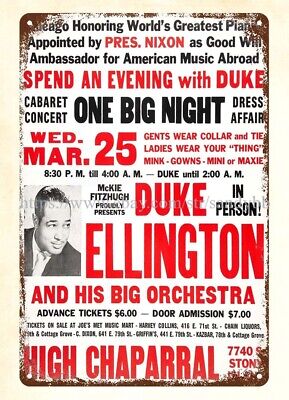The image features an old, rusted metal advertisement sign with a white background and various text in black and red. The sign is heavily rusted around the edges, particularly at the bottom, and each corner has a drilled hole. Dominating the sign is a promotion for a Duke Ellington concert, proudly presented by McKee Fitzhugh. The central headline in big black text reads "One Big Night," complemented by the red-lettered “Spend an Evening with Duke.” Additional text details the event as a "Cabaret Concert and Dress Affair," scheduled for "Wednesday, March 25th" from 8:30 p.m. until 4 a.m., with Duke performing until 2 a.m. The concert is to be held at the High Chaparral, 774 Stone Street. A photo of Duke Ellington, clean-cut with slicked-back hair, is prominently displayed in the center-left portion of the sign. The sign lists ticket prices as $6.00 in advance and $7.00 at the door, with tickets available at Joe's Music Hall. The attendees are advised on dress code: "Gents wear collar and tie. Ladies wear your thing. Mink gowns mini or maxi." Additionally, it mentions Duke Ellington being honored as the "world's greatest piano" and appointed by President Nixon as a goodwill ambassador for American music abroad.